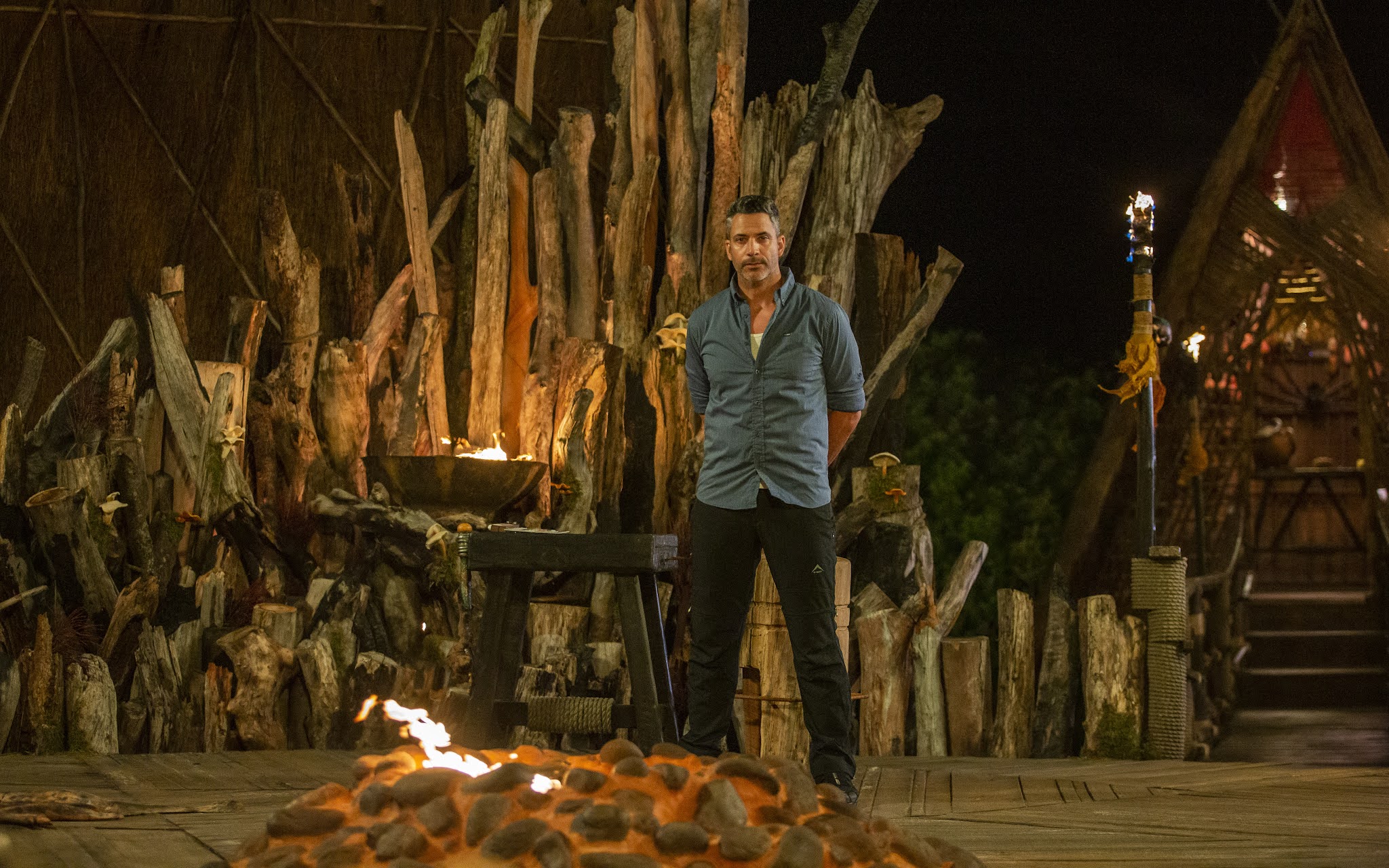In this evocative image reminiscent of a television set—possibly from a reality show like Survivor—a man stands at the center of a scene brimming with rustic, tropical elements under a black sky. The man, who appears to be the host, wears a blue-gray button-up shirt over a white t-shirt, paired with black pants. His dark hair and close-cropped beard, tinged with gray at the temples, add a rugged outdoorsy charm.

The foreground features a glowing rock fire pit emitting bright flames, surrounded by stones. Adjacent to it, there's a large, ornate pewter or copper bowl also ablaze. Slightly to the left, a small black stool stands unobtrusively. Vertical logs and sticks of various heights create a makeshift wooden fence behind the man, creating a natural backdrop.

To the right, there's a tiki torch adorned with raffia and an A-frame wooden hut elevated on a few steps, emanating a warm glow from within. The hut, with its V-shaped roof, suggests an indigenous or primitive design and houses a small table inside. Additional tiki torches and scattered pieces of wood enhance the scene, giving it a distinctly tropical island ambiance. The entire setup rests on a wooden platform or patio, contributing to the structured yet wild aesthetic of the portrayed environment.